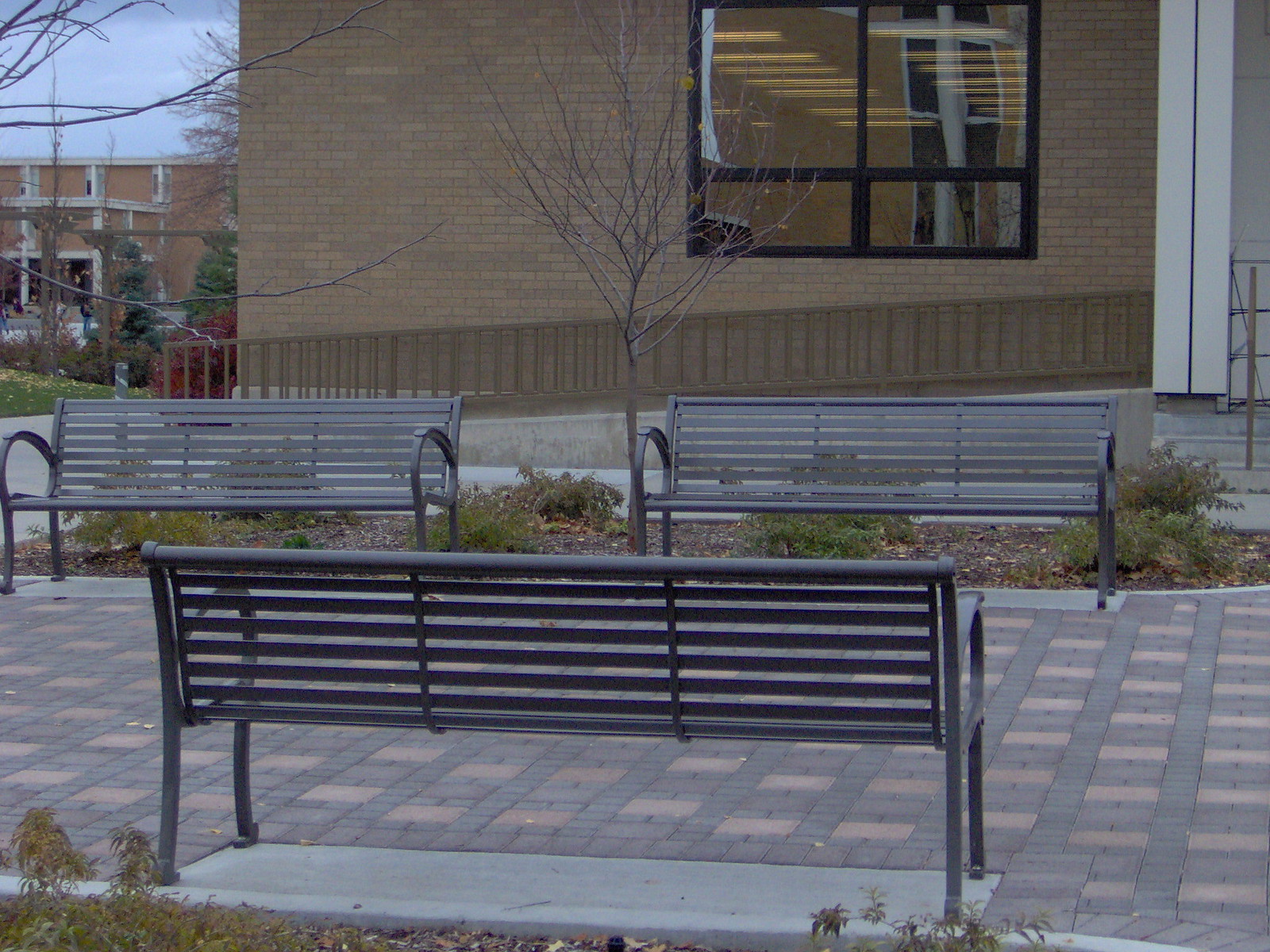In the early morning or evening light, a photograph captures three metal park benches on a neatly paved path made of grey and pale red terracotta colored bricks. Two benches face towards the viewer, separated by a small, bare tree, while a third bench, facing away, is in the foreground. Each bench sits on its own cement pad, enhancing their grounded presence in the scene. Flanking the benches are cheerful flower beds with shrubs.

Behind the benches, a beige brick building, potentially a school or a university, stretches across the background. The building features a large black-framed window, through which strip lights are visible, indicative of a commercial or institutional setting. A beige ramp with a handrail runs from right to left, providing wheelchair access. Toward the top right corner of the image, a staircase with a handrail leads upwards.

The sky in the top left corner is overcast with shades of grey, suggesting imminent rain or snow, adding to the wintery feel of the scene. Dry, leafless trees and distant evergreens are visible, contributing to the somber yet serene atmosphere. Another building can be seen further back on the left side, hinting at an extended campus area.